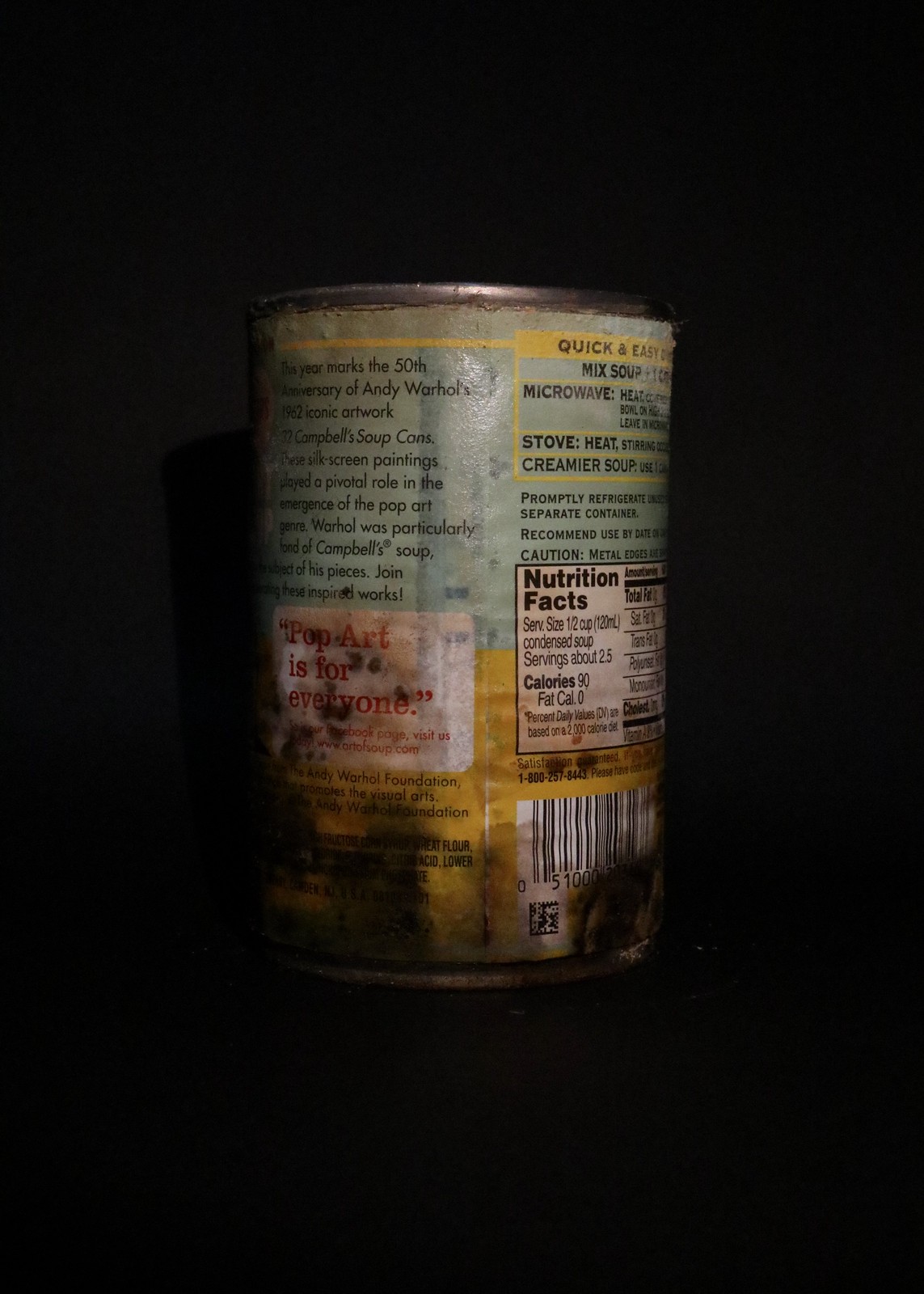The image showcases an old, weathered can centrally positioned against a solid black rectangular background. The can's label exhibits significant signs of age and wear, particularly noticeable by the blotchy blackened areas at the bottom. While viewing the rear side of the can, a partial barcode is visible in the lower right corner. Directly above the barcode is a nutrition facts label, and further up are incompletely visible directions. On the left side of the can, there's additional text, including a white label with the phrase "Pop art is for everyone." Beneath this label, there's faded black writing obscured by the darker patches on the can. At the top of the label, partially legible text reads: "This year marks the 50th anniversary of Andy Warhol's artwork. Campbell Soup. C-O-N-S. Silk Screen Painting. A pivotal role in the emergence of pop art. Andy Warhol was particularly fond of Campbell Soup. His pieces," followed by an unreadable section.